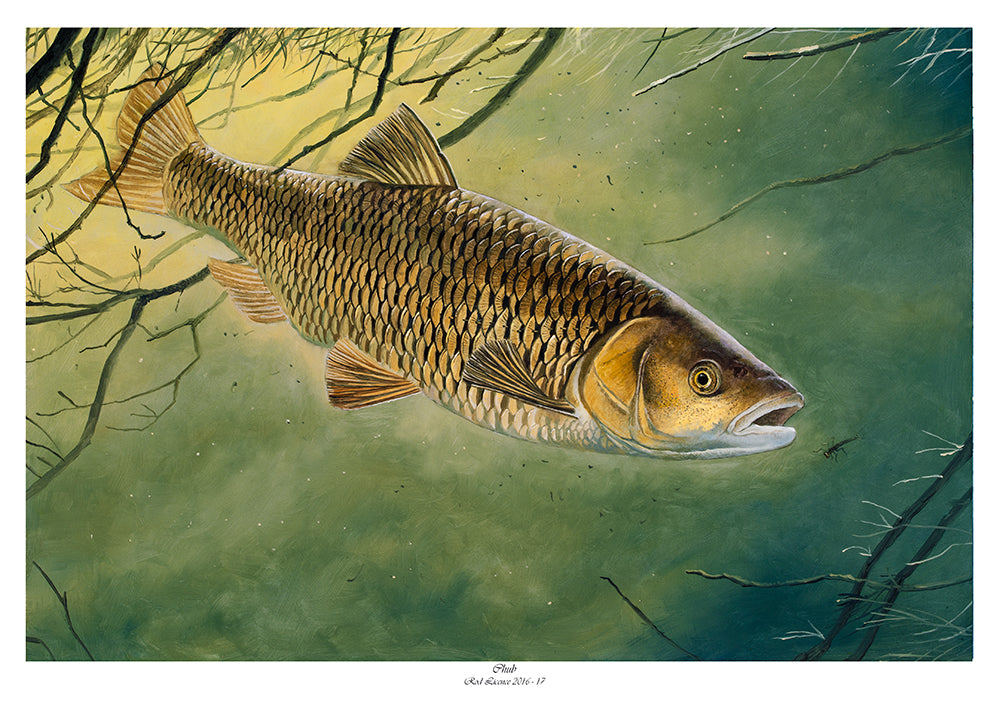This is a detailed watercolor painting of a large, golden fish, possibly a trout, amidst a lush aquatic setting. The fish, predominantly gold with a shimmery, scaly texture and accented with hues of pink and white, has four distinct fins. Its eye is a prominent black, encircled by rings of gold, sandy color, and brown. The head of the fish is notably gold.

The fish is depicted swimming through branches and roots of water plants, seemingly pursuing a small insect. The insect appears to be the fish's intended prey, adding a dynamic element to the scene. The background water is rich with shades of green, reflecting hints of blue from the sky above, enhanced by a golden grainy texture.

Beneath this vivid portrayal, there is a name inscribed, somewhat legible as starting with "P-L" and containing sequences like "R-A-L" and possibly "P-L-E-O". The signature includes the years "2016 to 2017", suggesting the period during which the artwork was created.